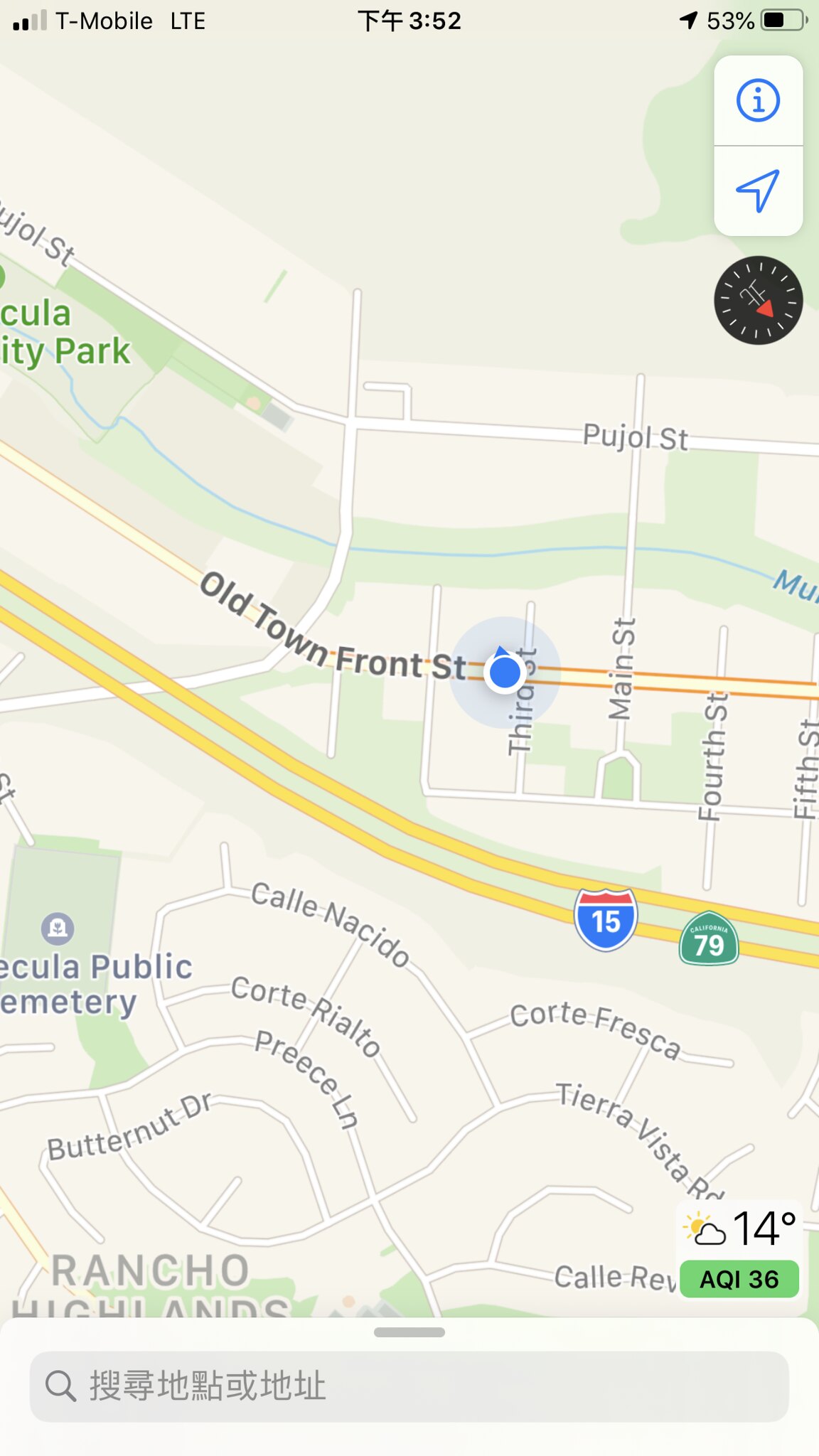**Detailed Caption:**

The image appears to be a screenshot of a Google Maps interface displayed on a smartphone. The map has a standard light gray background, with various areas shaded in slightly darker gray and different hues of mossy green to denote terrain and land usage. At the top of the screen, the phone's status bar indicates a T-Mobile LTE connection with two bars of signal strength. To the right, the battery icon shows a 53% remaining charge.

In the top middle section of the screen, a couple of Asian characters are displayed, possibly representing the location's language settings, alongside the number "352." An arrow symbol for map navigation appears adjacent to this. Toward the top right corner, an eye icon is visible for additional information options, along with another arrow icon whose function is unclear from this context. A small compass icon is also present for orientation purposes.

The map prominently displays "Old Town Front Street," indicating the user's or primary point of interest's location. The map also features two yellow lines marking Highway 15, alongside a sign indicating the 79 highways. Surrounding this area are various streets and landmarks, some of which have names partially or entirely visible. These include Main Street, 4th Street, 5th Street, Calina City, Nesito, Corte Fresca, Butternut Drive, Tierra Vista, and Rancho Highlands. Additionally, a city park is suggested by certain green areas, though not all names and details are fully readable due to display limitations.